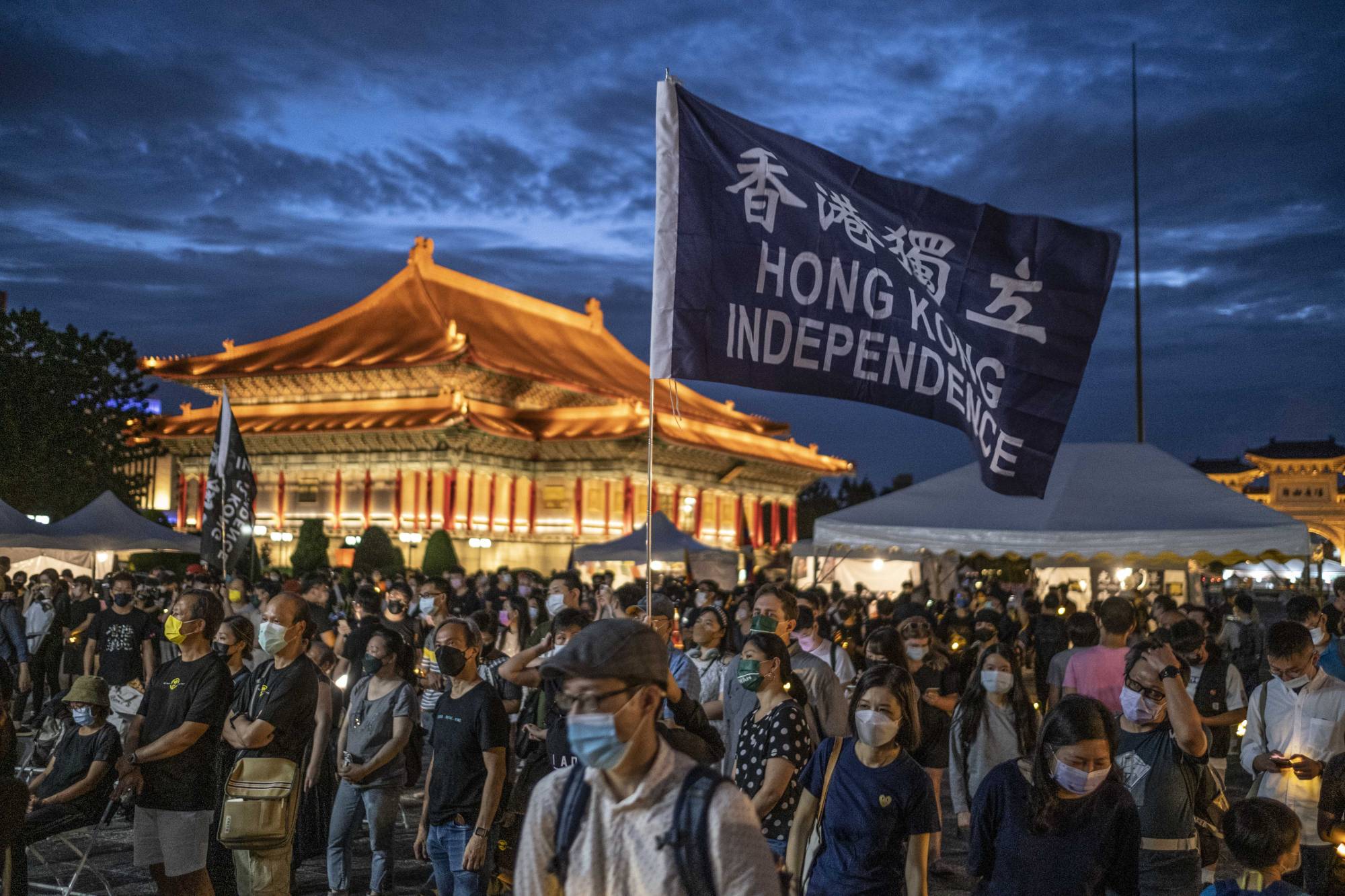The photograph captures a nighttime celebration featuring a massive crowd of hundreds of masked individuals, all seemingly of Asian descent, gathered at an event. Central to the scene is a prominent flag waving in the air, boldly inscribed with "Hong Kong Independence." The crowd, adorned in masks of various colors, includes individuals engaging in different activities such as using their phones, watching something not visible in the image, and sitting down. To the left, a group of four people stand with their arms crossed, looking toward the left. The foreground features a circular, tent-like structure with a white roof, surrounded by several smaller white tents interspersed among the crowd. In the illuminated background stands a traditional Chinese-style building, characterized by its gold elements and red pillars, providing a stark contrast to the cloudy, dark sky painted with shades of blue.